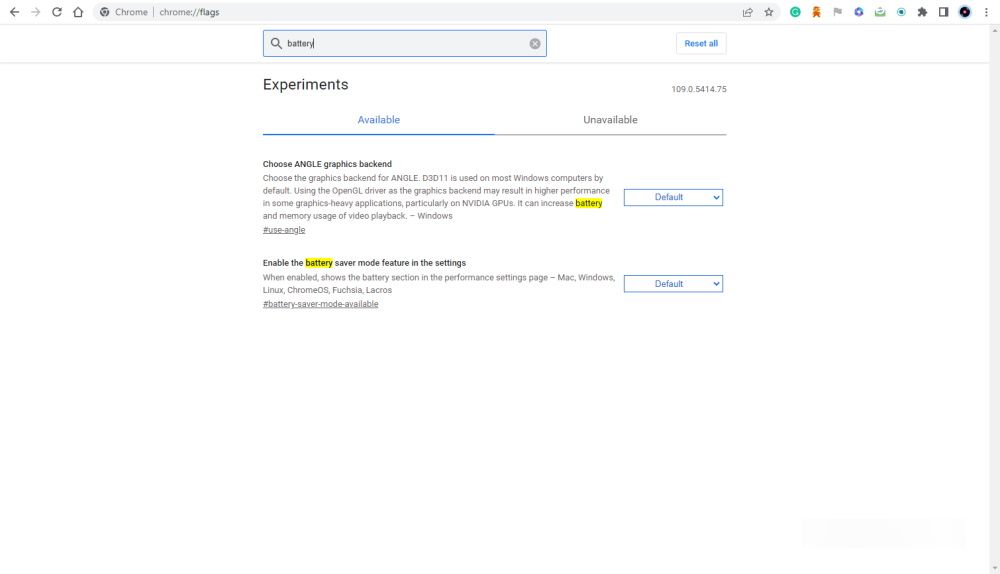This image is an edited screenshot of the Chrome browser displaying the "chrome://flags" settings panel. At the very top of the page is the primary search bar with the term "battery" typed into it. Adjacent to the search bar on the right, there is a "Reset all" button styled in a white background with blue text. Below the search bar, the word "Experiments" is displayed in bold black font.

The page is divided into two categories: "Available" and "Unavailable," with the "Available" category selected. Two options related to the search term "battery" are displayed under this category. 

The first option is labeled "Choose ANGLE graphics backend," accompanied by a brief description directly below it. In this description, the word "battery" is highlighted in yellow, indicating its relevance to the search query.

The second option is titled "Enable the Battery Saver mode in features and settings." This option also includes a short description with the term "battery" highlighted in yellow for relevance.

To the right of both options, there are drop-down menus, each set to "Default." The overall layout and highlighting effectively indicate that these settings are pertinent to battery-related functionalities within the browser.